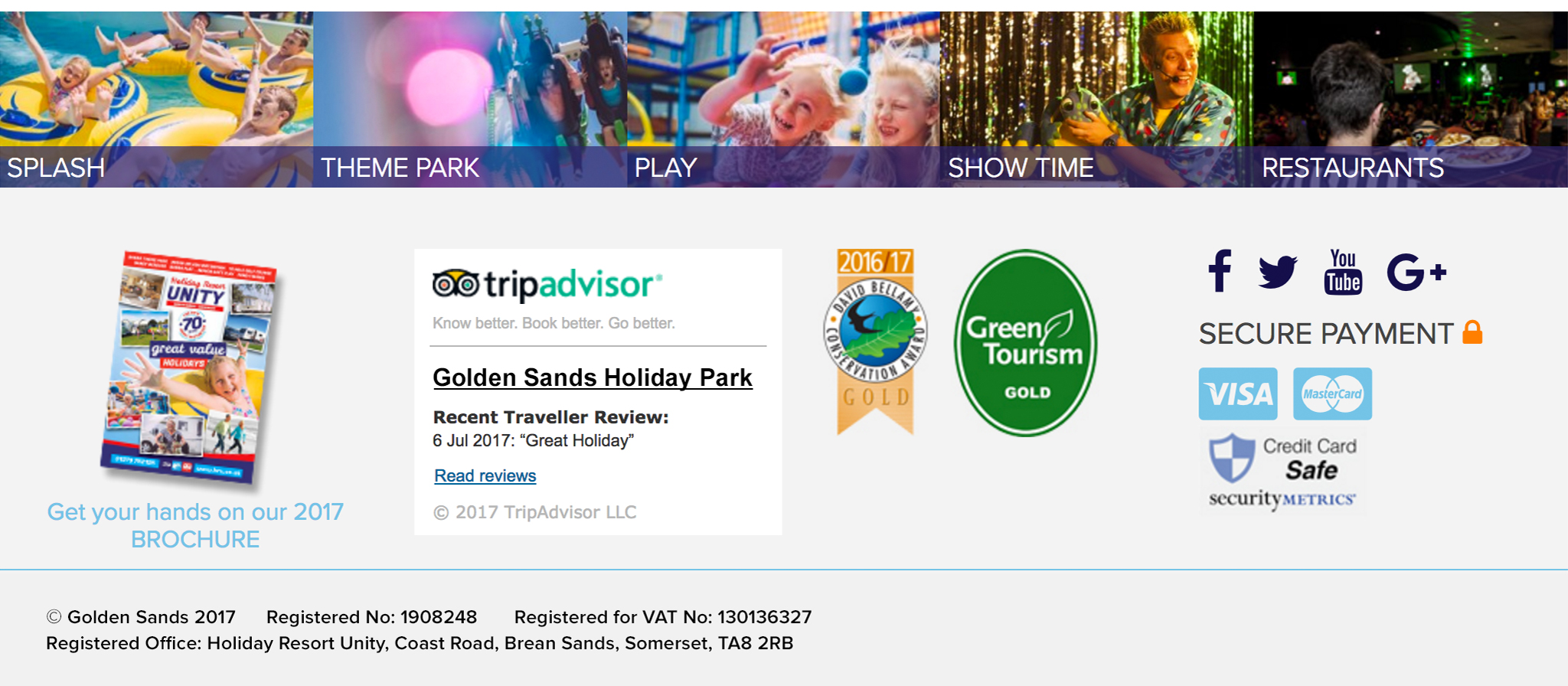This image is a cropped screenshot of an advertisement for Golden Sands Holiday Park. At the top of the screenshot, five photo thumbnails are horizontally aligned, each overlaid with a semi-transparent blue banner listing different activity categories. The first thumbnail shows people floating in inner tubes with the label "Splash." The second image depicts thrill-seekers on roller coasters, labeled "Theme Park." The third thumbnail features children playing, accompanied by the label "Play." The fourth presents a stage magician in action, titled "Showtime." Finally, the fifth image shows a person dining in a restaurant, labeled "Restaurants."

Below these thumbnails, the main body of the advertisement has a grey background. On the far left, a magazine cover is angled and centered above the text "Get Your Hands On Our 2017 Brochure" in prominent blue letters. The center section features a large white box displaying the TripAdvisor logo, followed by "Golden Sands Holiday Park Recent Traveler Review," a date, and a review titled "Great Holiday." Beneath this, a hyperlink labeled "Read Reviews" is present.

To the right, two awards are displayed: a green oval reading "Green Tourism Gold" and a conservation logo with an Earth emblem. Adjacent to these, a series of social media icons for Facebook, Twitter, YouTube, and Google+ are displayed. Further down, the text "Secure Payment" in bold grey is positioned next to a gold lock icon, with Visa and MasterCard logos beneath it. Centered at the bottom, a shield icon is followed by the text "Credit Card Safe."